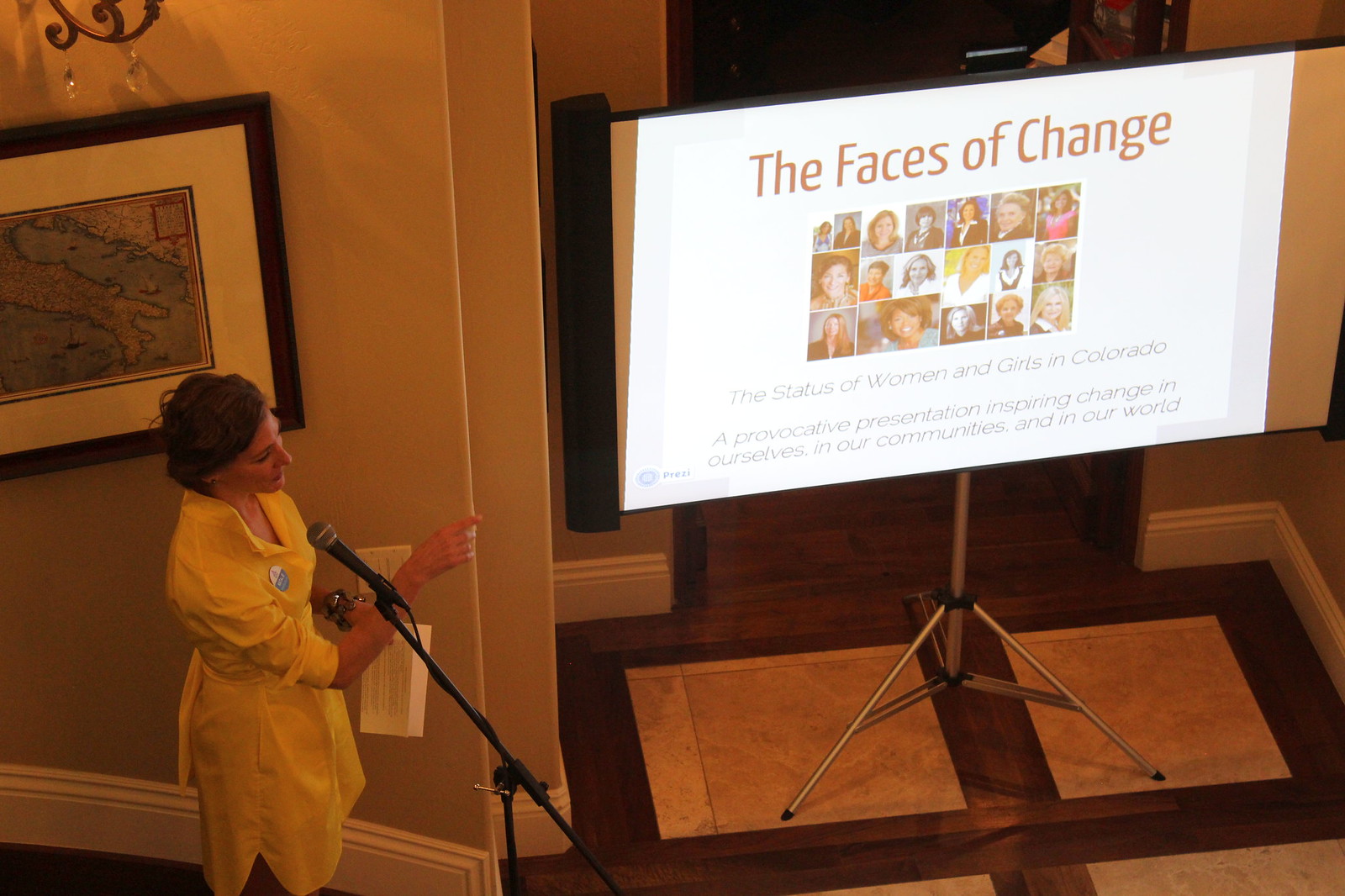The image depicts a top-down view, possibly taken from an elevated balcony or staircase, of a woman giving a presentation in an indoor reception room. Dressed in a light-colored, business-casual dress, she has a lighter skin complexion and short dark hair. The woman stands behind a microphone mounted on a black stand, and she is pointing to her right towards a projector screen. The large screen displays the title "The Faces of Change: The Status of Women and Girls in Colorado," along with the tagline "A Provocative Presentation Inspiring Change in Ourselves, in Our Communities, and in Our World," and shows a collage of faces. The background includes a framed picture, possibly an old map of Italy. The overall image is quite dark, and the woman’s gaze is directed towards the right, adding emphasis to the presentation slide she’s gesturing towards. This appears to be a detailed and evocative event centered around the theme of women and change.